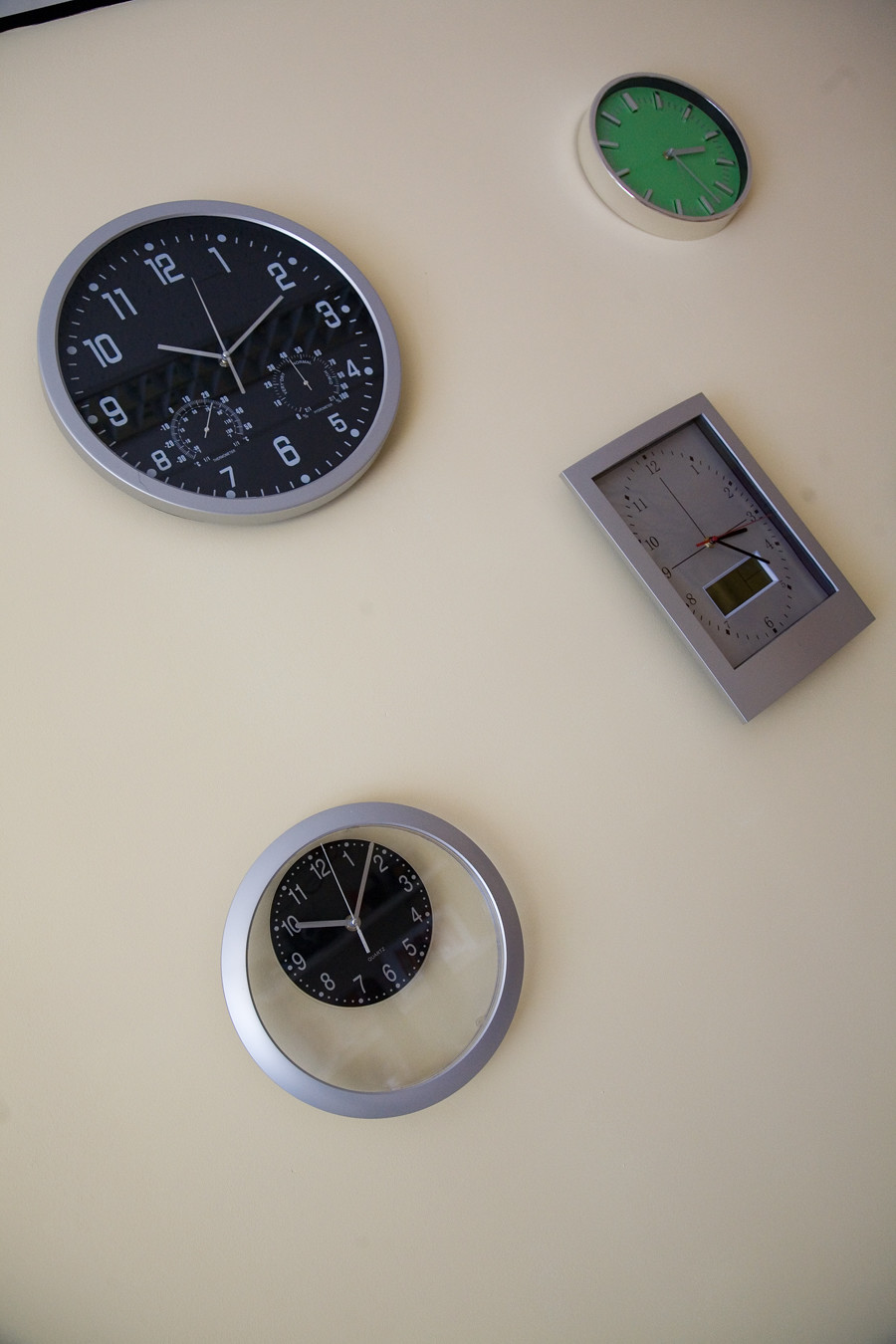The image features a creatively angled photo of a stark white wall adorned with four distinct clocks, each meticulously designed. Positioned slightly right and upward due to the tilt of the camera, the clocks present an intriguing visual arrangement.

- The clock on the far left stands out with its black face and silver rim. It is adorned with white hands and white numerals, including two smaller subsidiary dials at the center for additional timekeeping functions.

- To its immediate right, a clock showcases a green face contrasted by silver hands and hour markers, which are represented as lines rather than numbers. This piece is also encased in a silver frame.

- Below and slightly left of this clock, a vertically oriented rectangular timepiece features a monotone gray face and body. This clock is equipped with black hour and minute hands, complemented by a vibrant red second hand.

- Positioned further down and to the left, the final clock has a classic black face with white numerals and white hands. It is uniquely encased beneath a slightly larger protective glass cover with a silver trim.

All these timepieces are affixed to a pristine, completely white wall, enhancing their varied designs and creating a striking visual impact through their contrast.